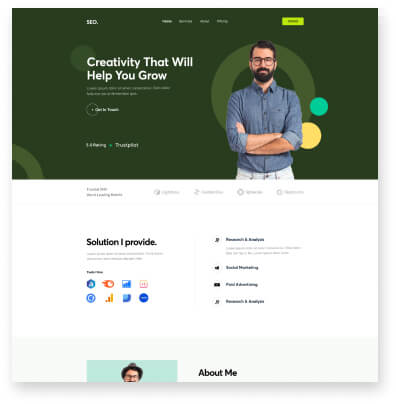A website with an olive green background features a central header with the text "HD" prominently displayed. Just below the header, in the middle of the page, the tagline "Creativity That Will Help You Grow" is visible. A man dressed in a long-sleeve blue button-down shirt and light blue pants stands centrally, framed by overlapping circles in various colors, including green, yellow, and turquoise.

A bright chartreuse button is located in the top right corner, drawing attention against the darker background. Beneath the main section, there are some navigation links on a white background, but they are illegible due to low resolution. Towards the bottom of the webpage, there is a smaller photo of possibly the same man, now wearing a hat, the area is labeled "About Me" on the right. The overall color scheme includes shades of olive green, light olive green, chartreuse, turquoise, and yellow, with text mostly in white.